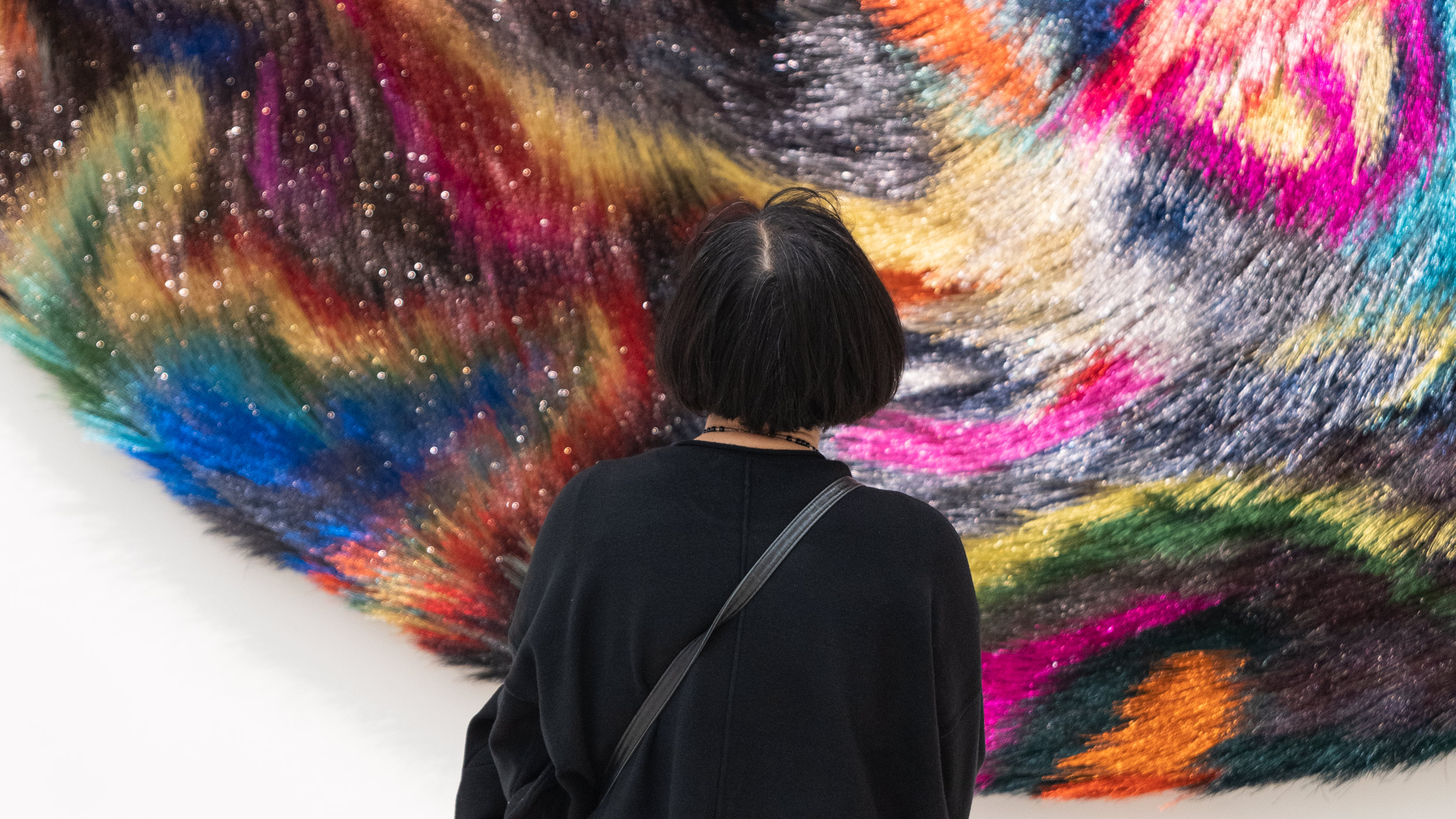In this color photograph taken in landscape orientation, the central subject is a woman standing in an art gallery with her back facing the viewer. She has short black hair and is wearing a black dress paired with a black cross-shoulder sling bag. Adding to her attire, she dons a black beaded necklace. The woman is intently gazing at a striking, three-dimensional exhibit displayed on a white wall in front of her. 

The artwork, a creation by artist Nick Cave, is part of a multi-medium installation at the Guggenheim Museum. It features a circular configuration with a furry texture and glitter, showcasing a rich array of swirling colors including various shades of blue, green, red, pink, yellow, gray, brown, and purple. This colorful piece spans nearly the entire width of the photograph, leaving only a small portion of the white wall visible in the bottom left corner. The vibrant feathers or hair-like textures create a visually captivating pattern that draws the viewer's eye, embodying a style that blends photographic representationalism with realism.